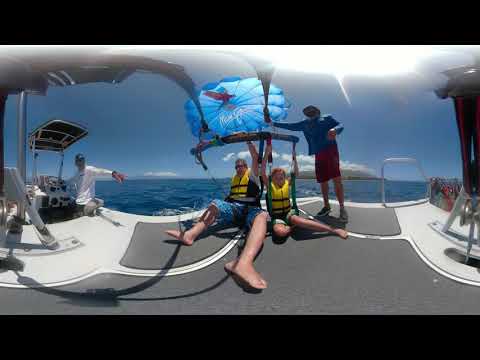The image depicts a group of individuals on the back deck of a boat, clearly prepared for a parasailing adventure. The scene is bordered by thick black edges on the top and bottom of the picture, adding a dramatic frame to the vibrant activity. At the center of the image, a man and a woman sit side by side in yellow life vests, facing forward. Both are dressed in shorts without shoes; the man, positioned on the left, has his legs stretched out in front, his left leg notably distorted and elongated due to the angle. The woman, on the right, has her right leg bent back and her left extended outward. They appear poised for their parasailing experience, the deck beneath them a mix of gritty tarmac and white enamel surfaces designed for safety and grip.

Above these seated individuals is a blue parasail, partially visible and likely connected to a harness system suggested by the ropes and equipment hanging above them. To their left, an individual in a long-sleeved white shirt appears to be gesturing, possibly managing the boat's controls at a nearby panel. On the right stands another person involved in the activity, identifiable by his blue shirt, red shorts, and a hat. He has something in his left hand while his right hand interacts with the parasailing gear above the seated duo. The scene behind includes a broad expanse of calm, royal blue water, hinting at an ocean or large lake setting, bathed in bright sunlight with a nearly cloudless sky, except for a few clouds on the distant horizon. Various structural elements of the boat are faintly visible, including a railing and possibly the cabin on the far right side of the frame.